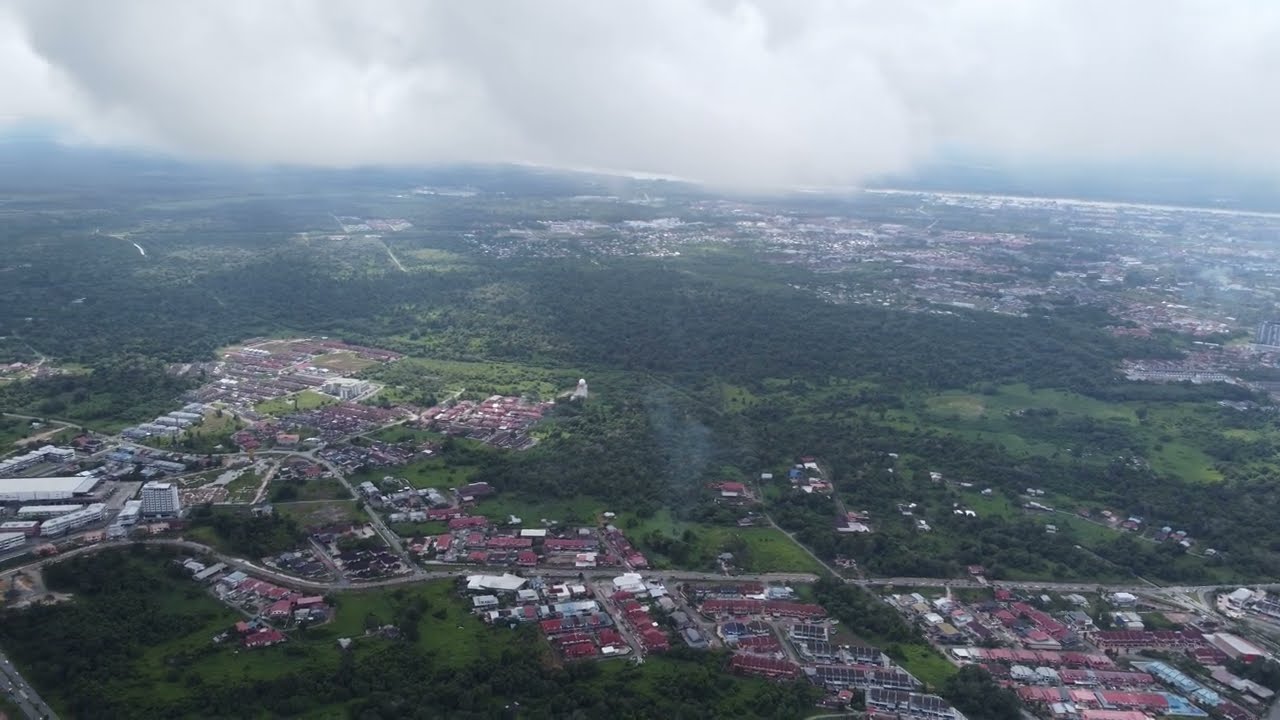This is a detailed aerial color photograph, likely taken from a drone or a high vantage point, capturing a suburban town or village with a mix of housing, greenery, and roadways. The overall scene is fairly balanced between structures and natural elements, with possibly slightly more green space than built-up areas. The majority of the buildings are residential with red tile roofs, predominantly limited to two or three stories. Roads wind through the scene, with some vehicles visible but no discernible individual people due to the high altitude of the photograph. The bottom left features farmland, transitioning into suburban housing which greatly populates the right and top right sections of the image. The middle region is characterized by a blend of farmland, trees, and forested areas. In the background, a pale blue mountain range is visible in the top right, partially shrouded by clouds that linger overhead. Overall, the photograph embodies a realistic, representational style of a peaceful, verdant suburban area interspersed with pockets of urban development.